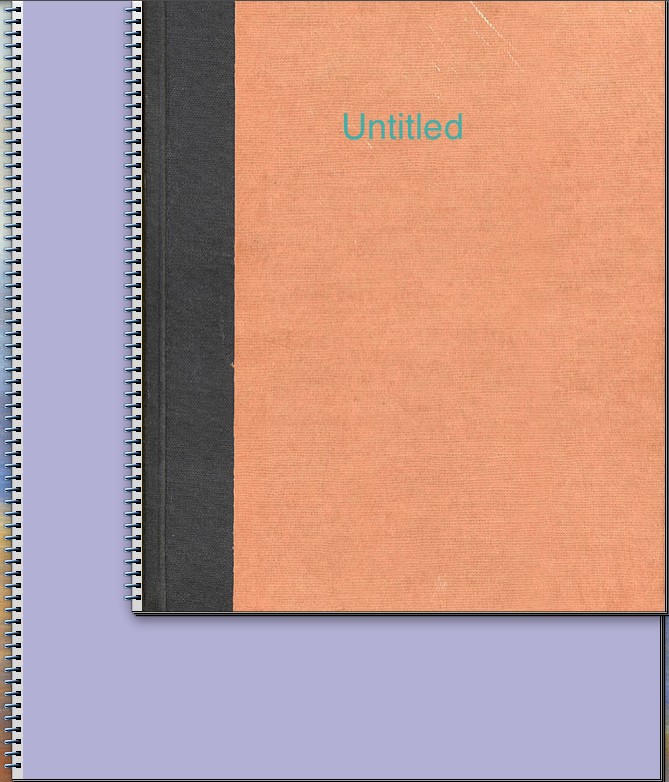This colored image features two spiral-bound notebooks against a plain, seamless background. The larger notebook, positioned at the back, has a smooth, light purple cover with no visible text. The smaller notebook is resting on the top right corner of the larger one and is slightly more intricate in design. It boasts a rust-colored cover with a black spine, where the metal spirals are situated. There is notable texture on this cover, highlighting its durable construction. In the center of the smaller notebook's cover, the word "Untitled" is printed in gray lettering. Overall, the image captures the contrast between the plain, smooth purple notebook and the textured, more robust brown notebook, creating a simple yet striking composition.